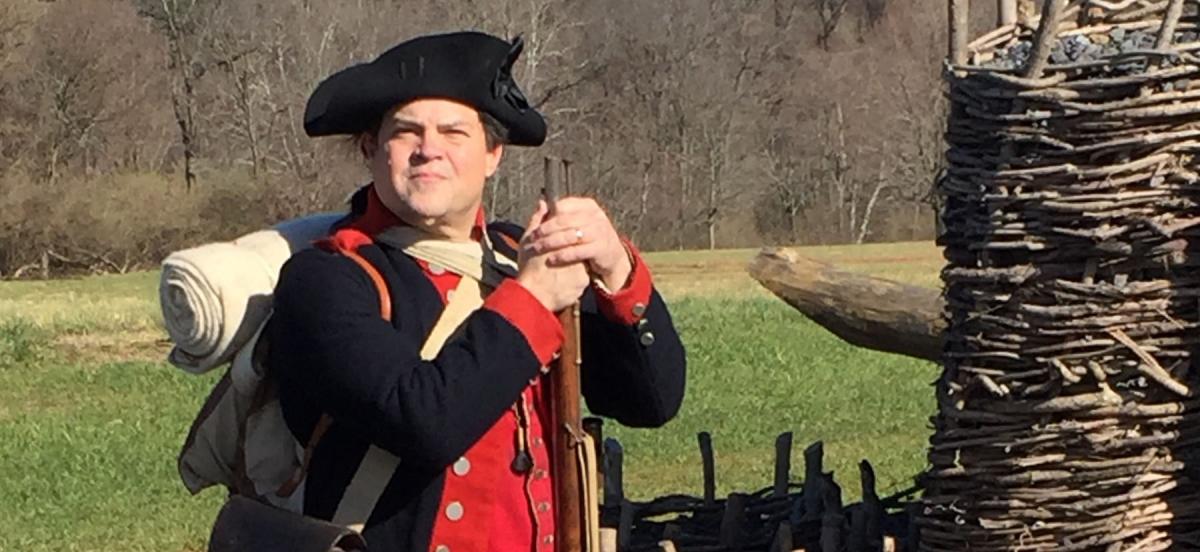A highly detailed scene set in an outdoor landscape unfolds before us. Central to the image is a middle-aged man who stands in the center-left of the frame. He is turned slightly, with his body angled at approximately the five o'clock position, giving focus to his face. This man wears an outfit reminiscent of a colonial or Civil War soldier. His attire is quite distinctive: a black colonial hat rests upon his head, and he is clothed in a black coat with red cuffs and a red button-up shirt adorned with silver studs down the front. His coat sleeves also feature buttons and cufflinks. He has a white backpack strapped securely on his back, from which a rolled-up item, likely a sleeping bag, is visible. 

The man is holding a tall gun with both hands placed near the top at the barrel. This gun's frame is brown, while the barrel itself appears blackish in color. 

Surrounding him, there’s a vividly detailed backdrop featuring elements indicating a wintry scene. Bare trees devoid of leaves stand in the background, suggesting the time of year. Additionally, green grass interspersed with patches of brown, bare land contributes to this seasonal hint. To the right of the man, there is a structure composed of wooden sticks, resembling a fence or perhaps a rudimentary shelter framework. Adjacent to this is a wooden log or pole. A bush is visible on the far left side of the image, aiding in framing the scene within this natural, sunlit setting.